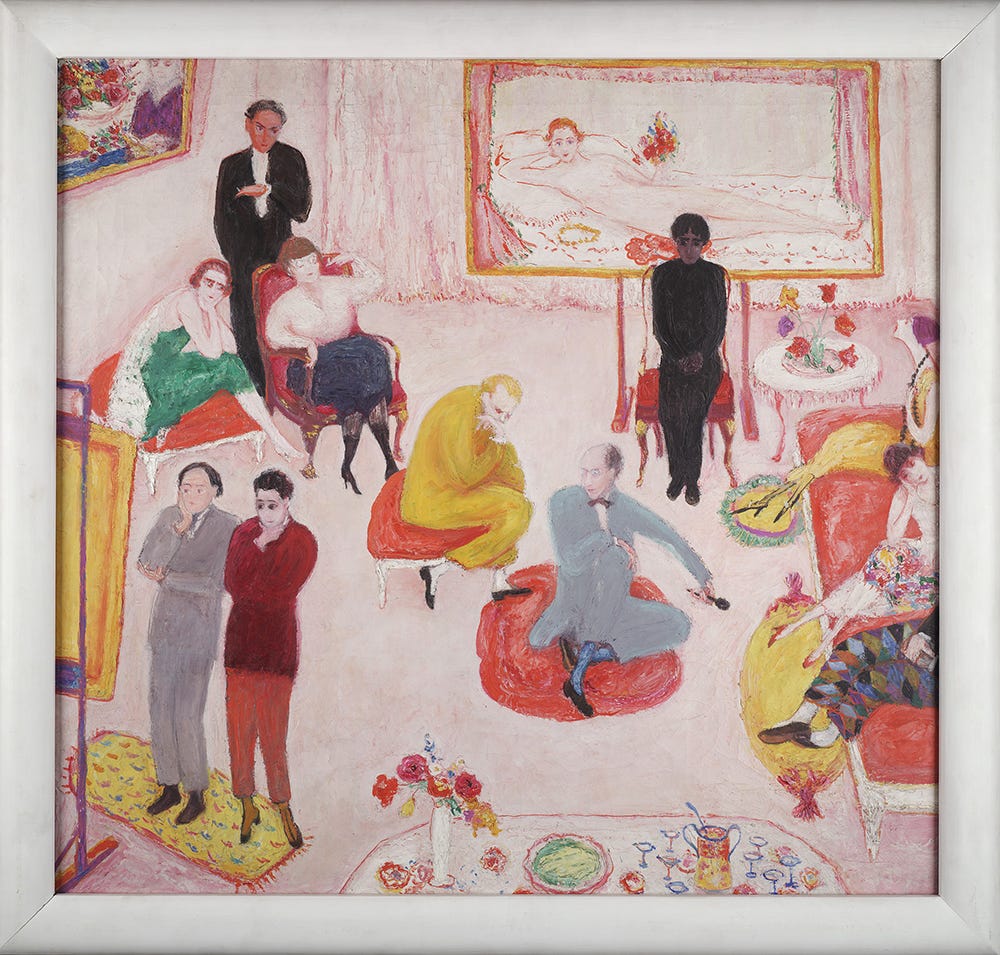The image is an intricately detailed sketch-like painting set in what appears to be a 1920s or 1930s art gallery or a sophisticated living room filled with an eclectic mix of people engaged in various activities. The room is characterized by dominant colors of red, yellow, and whitish hues. 

In the background, a framed painting of a naked woman lying on a bed is prominently displayed on the back wall, hinting at an art-focused theme. Below this artwork, a woman in a black dress is seated on a red chair, adding a focal point to the composition.

In the midsection of the room, two red beanbag-like chairs are occupied by two men in gray suits. One man appears to be holding a microphone and has his legs crossed. Surrounding these central figures, multiple chairs and seating arrangements are scattered about, with numerous guests either seated or standing.

On the lower left side of the painting, two men are standing closely beside each other on top of a yellow rug, intently observing another piece of art which is set up on an easel. One of these men is distinguished by a red shirt and orange pants, while the other is in a suit.

To the far right, a long red couch accommodates three women, providing a sense of social interaction and leisure. Additional details include a man standing behind seated guests, possibly smoking a cigar, and various tables with displays of drinks and flowers, enhancing the communal and lively atmosphere of the scene.

This elaborate painting captures the essence of an art gallery or a refined social gathering from the early 20th century, filled with individuals dressed elegantly in suits and dresses, deeply engaged with the artistic surroundings.